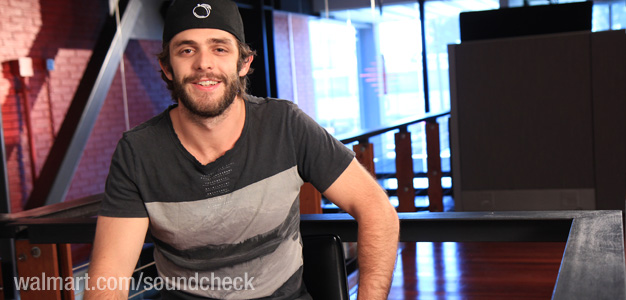In this detailed photographic image, taken indoors and watermarked in the lower left corner with "walmart.com/soundcheck," we see a young white man, likely in his twenties. He has dark, slightly unkempt hair that reaches over his ears, and he sports a black mustache and beard. He is wearing a black baseball cap backwards, featuring a white circular graphic, possibly resembling a ring or a peach logo, prominently on the front. His attire includes a t-shirt composed of dark and light gray sections.

Situated in front of what appears to be a studio setting, the young man stands slightly left of center, smiling at the camera. The background reveals a complex interior with several detailed elements: a brick wall with some panels and a girder to the left, and a polished wooden floor that adds warmth to the scene. There is also a staircase railing consisting of wooden posts and connecting boards. Further back, a stage setup is suggested by another railing, with large windows that allow light to stream through. These windows are blurred, obscuring the red words written on them. The mix of architectural features, such as the polished floor and large windows, coupled with the indistinct background details, creates a textured and dynamic atmosphere for the image.